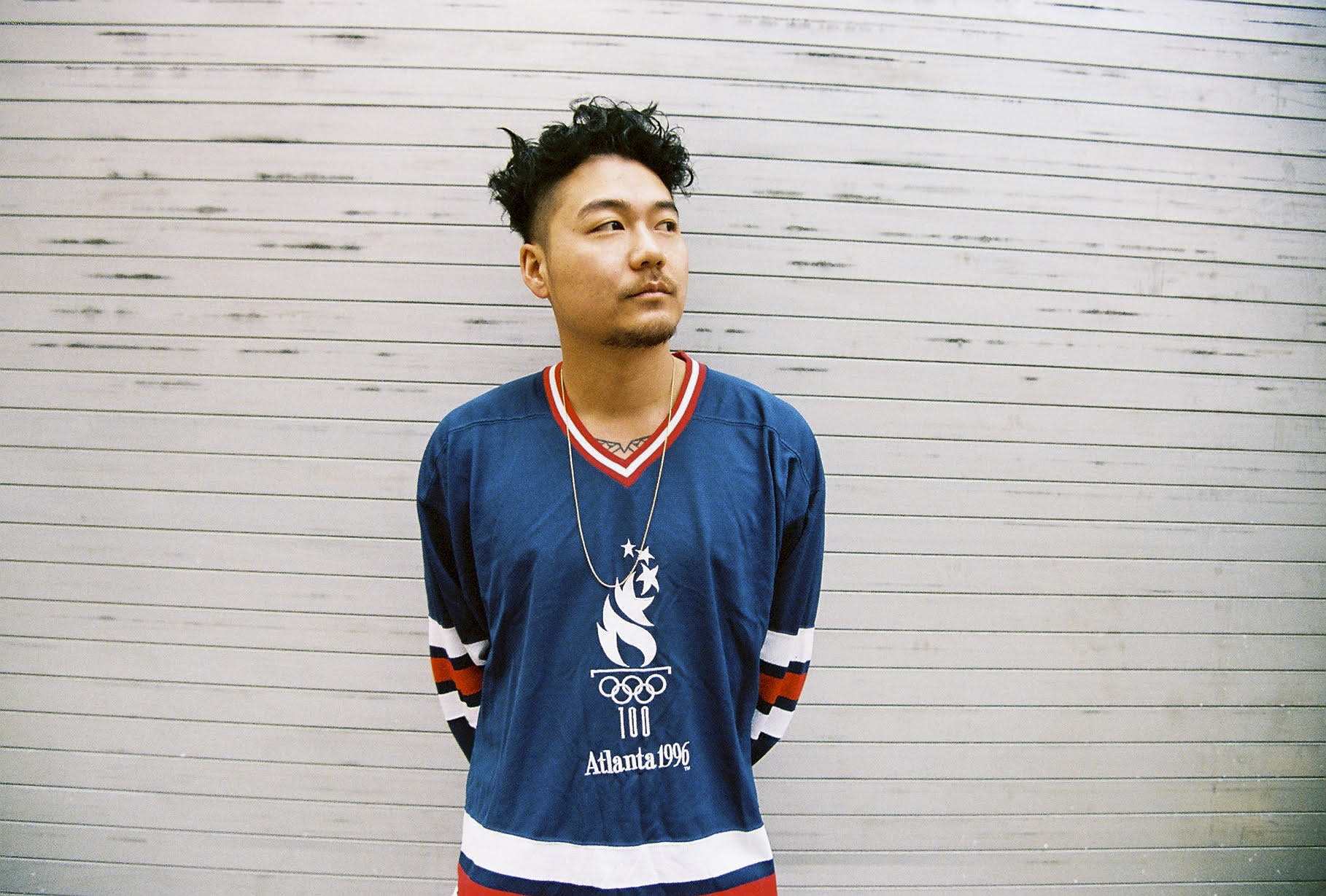A mid-shot image captures an Asian man standing and gazing thoughtfully to his left, our right. He has black hair styled neatly, complemented by a mustache and a goatee, and his black eyes reflect a neutral, serene expression. The man's attire is a blue shirt proudly emblazoned with the Atlanta 1996 Olympics logo, featuring the iconic Olympic torch above the five interlocking rings, all rendered in white. Below the logo is the inscription "100" and "Atlanta 1996." The shirt is distinctively designed with stripes of red and white on the collar, sleeves, and base. This characteristically vibrant attire stands out against the white painted wall behind him, likely made of wood or siding. The composition suggests an outdoor setting during daylight, even though the lower half of the man’s body is not visible. The backdrop, a plain white wall, serves to highlight the subject, making his features and clothing the focal point of the photograph.